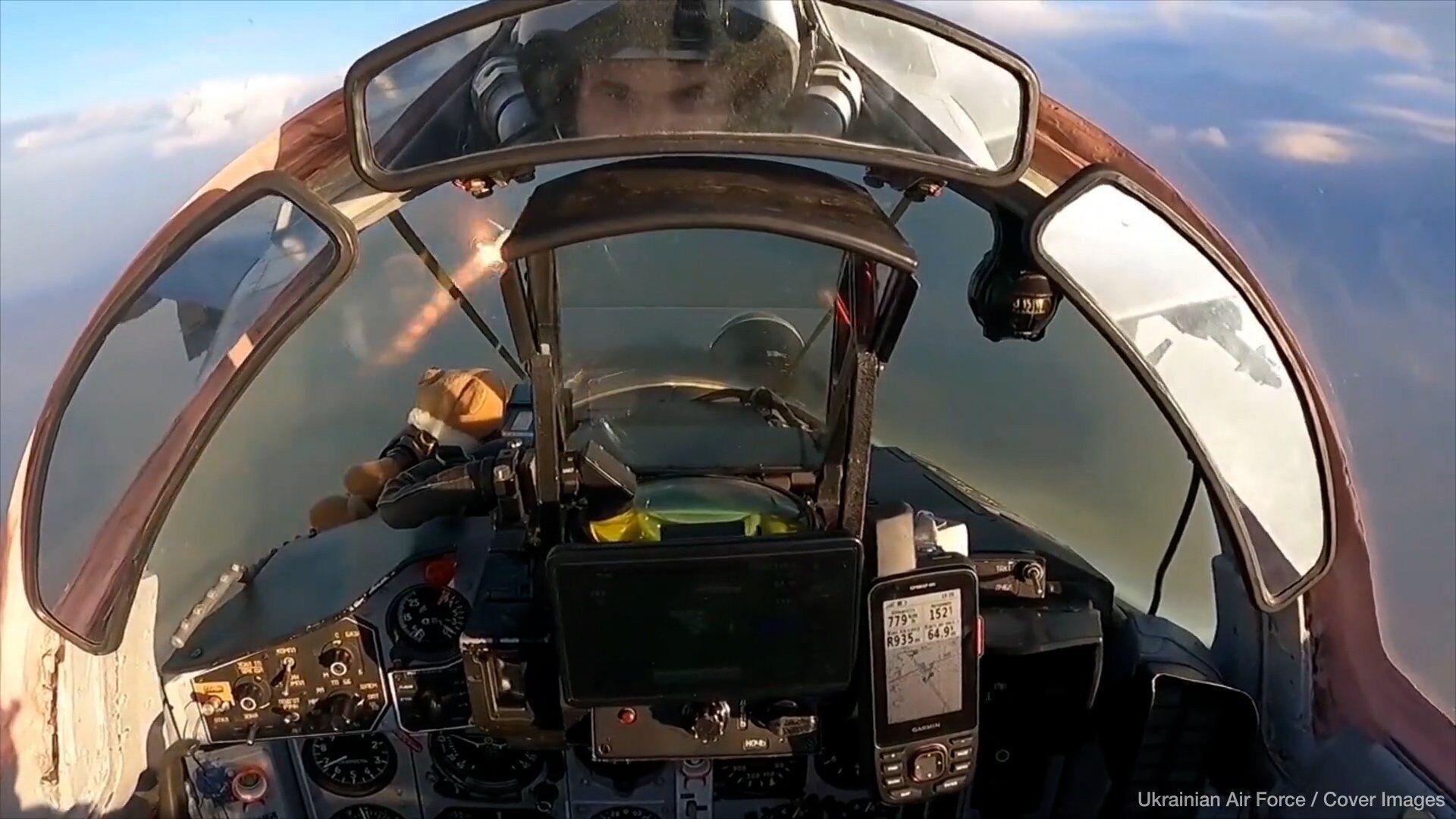This detailed color photograph, taken from within the cockpit of an Air Force jet soaring high in the clear daytime sky, captures an intense action shot featuring the Ukrainian Air Force. The cockpit is equipped with standard instrumentation, including an altimeter, airspeed indicator, and artificial horizon. On the right-hand side, a Garmin GPS unit is visibly affixed, likely secured in place. The transparent glass canopy allows for a panoramic view of the thin, sunlit clouds outside. At the top of the image, three mirrors are mounted, with the center mirror reflecting the pilot's face. The pilot, who may also be the photographer, sports a helmet that reveals only his dark eyes and brown eyebrows. Adding a touch of personal charm, a small teddy bear is seen in the cockpit, lending a sense of warmth to the high-stakes environment. The photo is marked in the bottom right corner with the text "Ukrainian Air Force / cover images," emphasizing its official and possibly published nature.